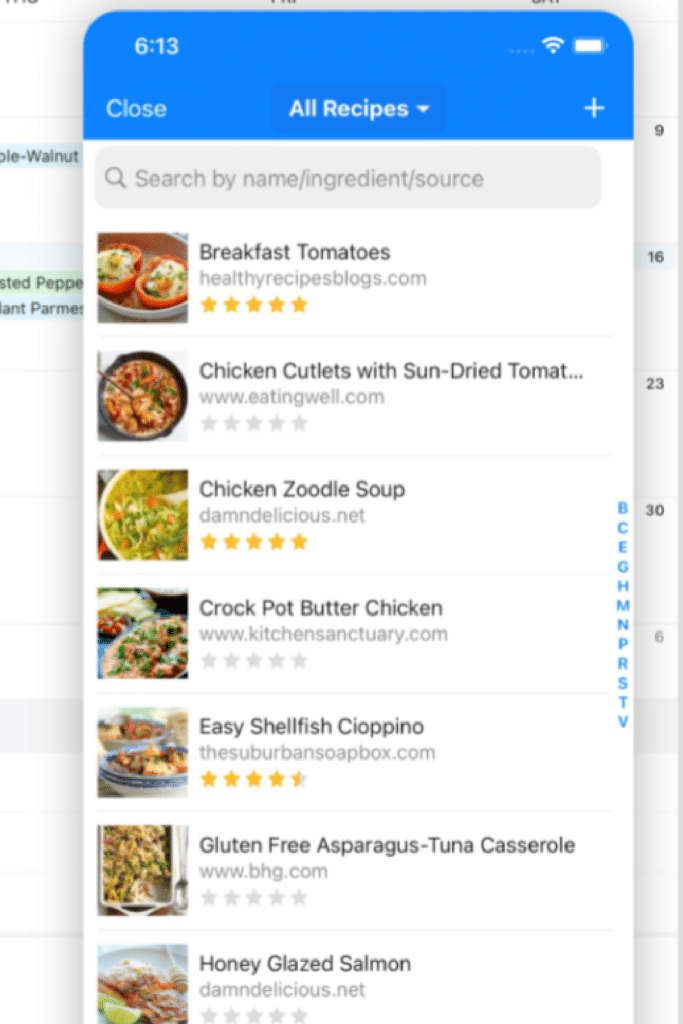This image depicts a meticulously layered screenshot configuration. The background is an edited screenshot of a recipe, partially visible to the left and right edges, with significant cropping on all sides, particularly on the bottom, revealing a gray bar where it was truncated. Overlaid onto this background is a mobile landscape screenshot from a recipe app. This app interface is bordered at the top by a distinctive blue strip featuring a centered drop-down menu labeled "All Recipes."

Beneath this header, the app presents its content on a clean, white background. At the very top of the app body, there is a search bar inviting users to find recipes by name, ingredient, or source. Directly below this search area is a vertical scroll list of seven recipes, each encapsulated within its own rectangular section.

Each recipe entry displays a small, square thumbnail image to the left, paired with the recipe's title in bold black font to the right. Directly under the title, the recipe source website is specified, and just below, a star rating is indicated. Here are the details of the first few recipes listed:

1. **Breakfast Tomatoes**
   - **Source:** healthyrecipesblogs.com
   - **Rating:** 5 stars

2. **Chicken Cutlets with Sun-Dried Tomatoes**
   - **Source:** eatingwell.com
   - **Rating:** No reviews (5 stars, all uncolored)

Subsequent recipes follow an identical layout, displaying their respective titles, source websites, and star ratings.